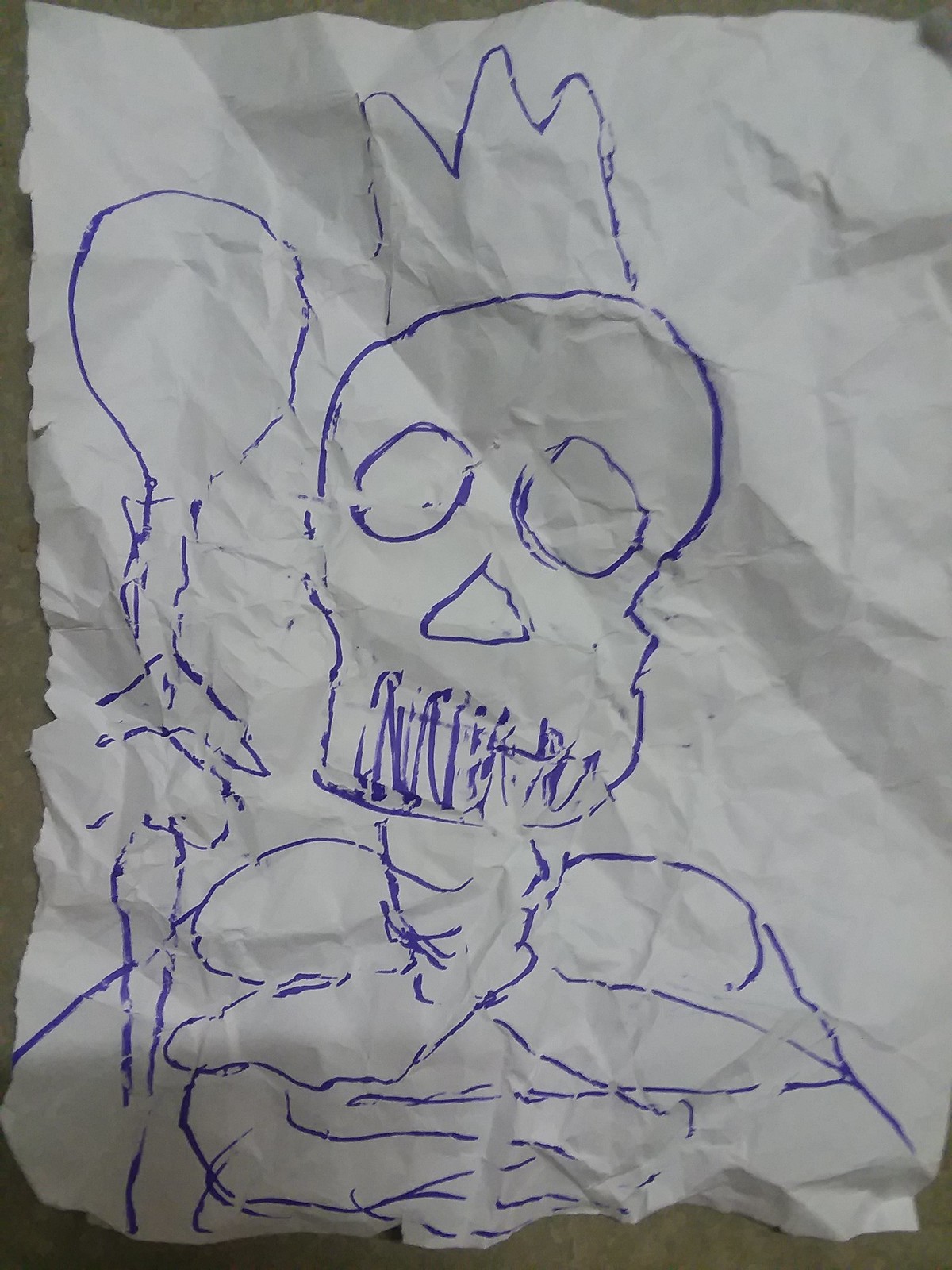This photograph captures a unique piece of artwork that was meticulously drawn on a white sheet of paper using a purple pen or marker. The drawing has been subjected to crumpling and squishing, then re-flattened, resulting in a multitude of shadows and creases that add depth and texture to the image. The central figure in the artwork is the outline of a skull's head, accompanied by the upper portion of a skeleton. The skeleton is adorned with a regal three-pointed crown and appears to be grasping a staff with a round tip, imbuing the illustration with a sense of authority and mystique.